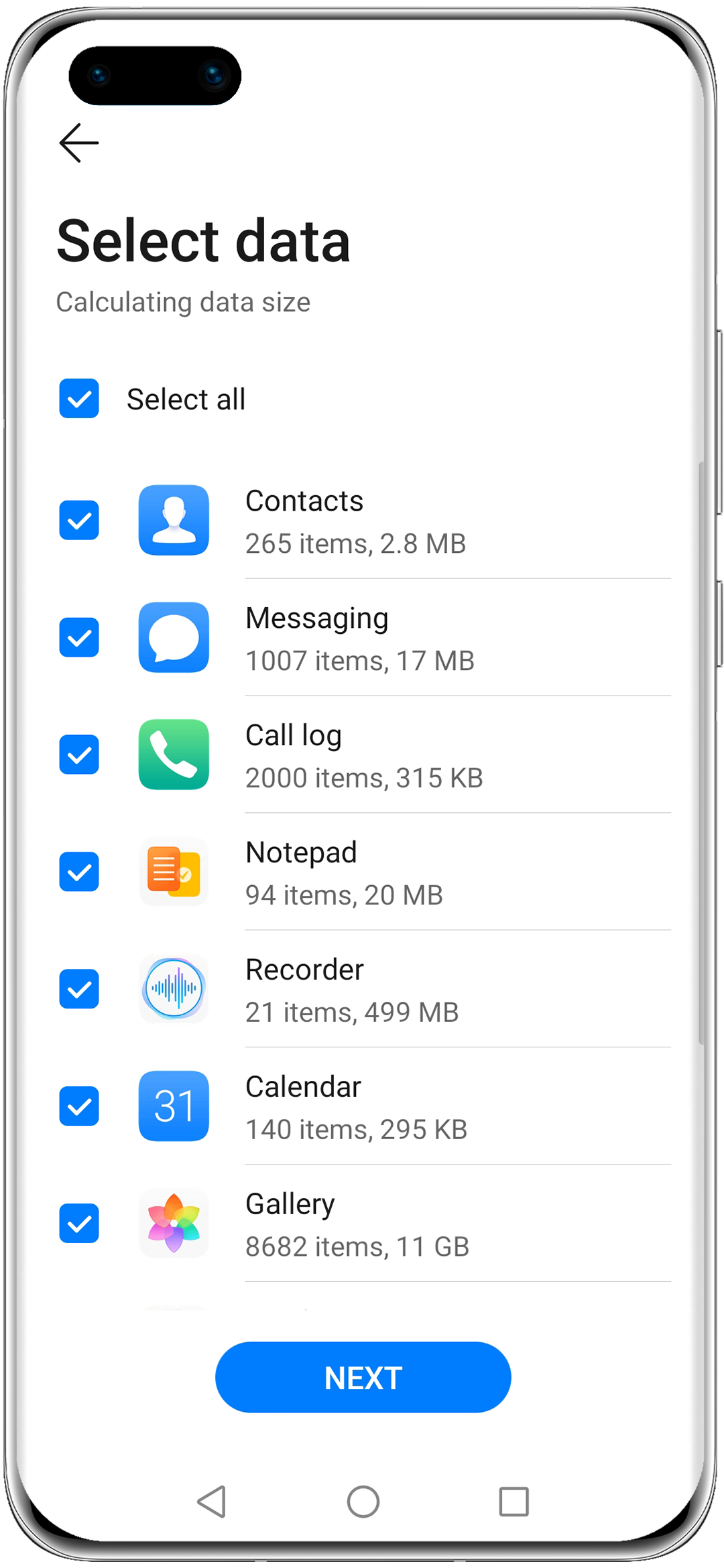The image depicts a smartphone without a protective case. On the device's right-hand side, there are two noticeable silver buttons. The phone display is active; the upper section of the screen is white with an oval element that houses two small camera lenses on either side, indicating a dual-camera setup.

Beneath this top section, the screen's content transitions to a black background featuring white text. The text is partially highlighted and reads, "Select Data," followed by "Calculating Data Size." A series of checkboxes are listed below, all marked with blue checks against white backgrounds, indicating selected items.

The first checkbox is labeled "Select All." Subsequent checkboxes include detailed data categories and their respective sizes:
- **Contacts:** 265 items, 2.8 MB
- **Messaging:** 1,007 items, 17 MB
- **Call Log:** 2,000 items, 315 KB
- **Notepad:** 94 items, 20 MB
- **Recorder:** 21 items, 499 MB
- **Calendar:** 140 items, 295 KB
- **Gallery:** 8,682 items, 11 GB

Each checkbox is separated by a thin gray line, clearly demarcating the different categories. The visual design conveys an organized and systematic approach to data management.